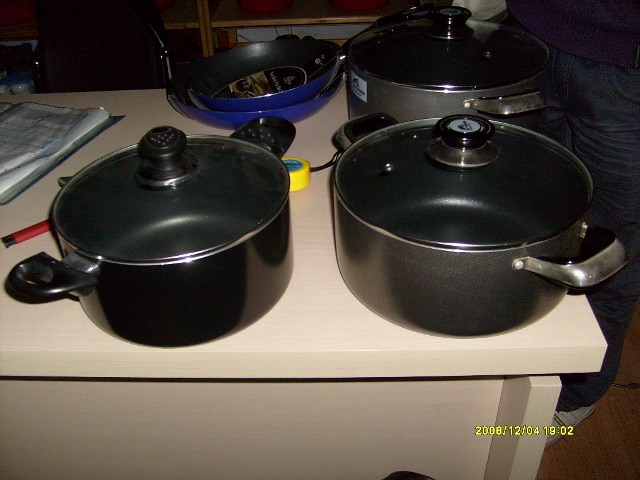This is a detailed photograph taken from above a kitchen island made of white particle board. The image features a variety of clean, empty cooking pots and pans, including three Dutch ovens or stockpots of different sizes, each with transparent lids featuring black handles and knobs. Additionally, there are two bright cobalt blue sauté pans with black interiors, neatly nested inside each other. The scene also includes a couple of woks and two spatulas. An open book, possibly a recipe book or paperwork, sits on the left side of the island, accompanied by a red disposable lighter. At the top right corner, a person is visible, wearing white sneakers, blue jeans, and a navy blue shirt. The photograph is date stamped 2008/12/04 and time stamped 19:02 in yellow at the lower right corner, marking when the picture was taken.